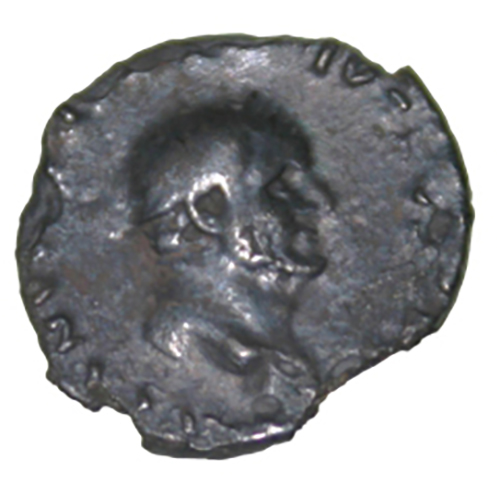The image features a severely damaged, deformed metallic coin set against a white background. The coin, possibly a nickel or a dime, appears old, with a dirty gray and brown coloration that reflects white light. The degradation is so extensive that the edges seem to have been slammed against a hard surface, creating indentations that obscure much of the text along the circumference. Though the symbols around the edge are mostly unrecognizable, a single character, a "2," is discernible on the left side. The most prominent feature of the coin is the engraving of a man facing to the right at the center, but the face is heavily distorted by indentations and dirt, making identification difficult. Overall, the coin's condition and the mysterious, partly obliterated inscriptions suggest a long history and significant wear.